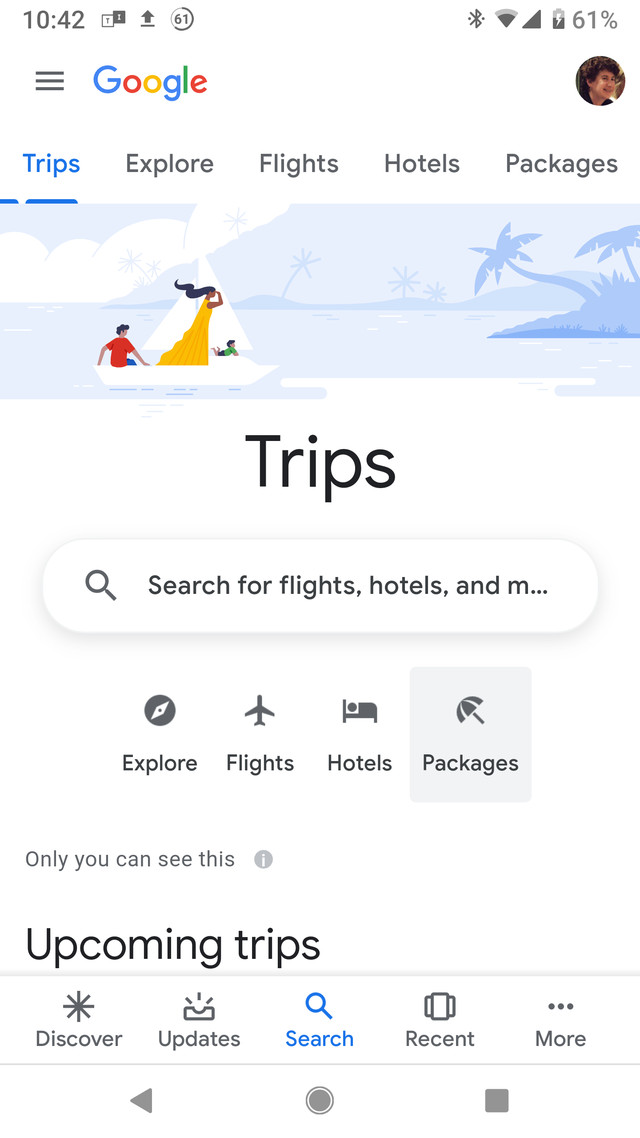The image depicts a vertically rectangular screenshot from a cell phone with a predominantly white background. At the top left corner, there is a dark gray bar displaying the time as 10:42, accompanied by multiple icons. On the top right, there are additional icons indicating Bluetooth, Wi-Fi, a signal bar, and a battery level at 61%.

Below this status bar, on the left side, there are three horizontal bars representing the menu icon. To its right, the Google logo is prominently displayed, and farther to the right is a small avatar circle featuring a face, though the details are too small to discern clearly.

Directly below the Google logo, there is a navigation bar. The first item, "Trips," is highlighted in blue with an underline, while the other items — "Explore," "Flights," "Hotels," and "Packages" — are presented in dark gray. Underneath this navigation bar, there is a simple illustration of three people in a sailboat heading towards an island on the right side of the image.

Centered beneath the illustration in large lettering is the word "Trips." A search field is located below this title. The navigation bar is replicated below the search field, with the "Packages" icon highlighted against a light gray background, indicating it has been selected.

Further down, a message reads "Only you can see this." Following this, the bold heading "Upcoming Trips" is prominently displayed. At the very bottom of the image, there is another row of icons labeled "Discover," "Updates," "Search" (highlighted in blue), "Recent," and "More," offering additional navigation options.